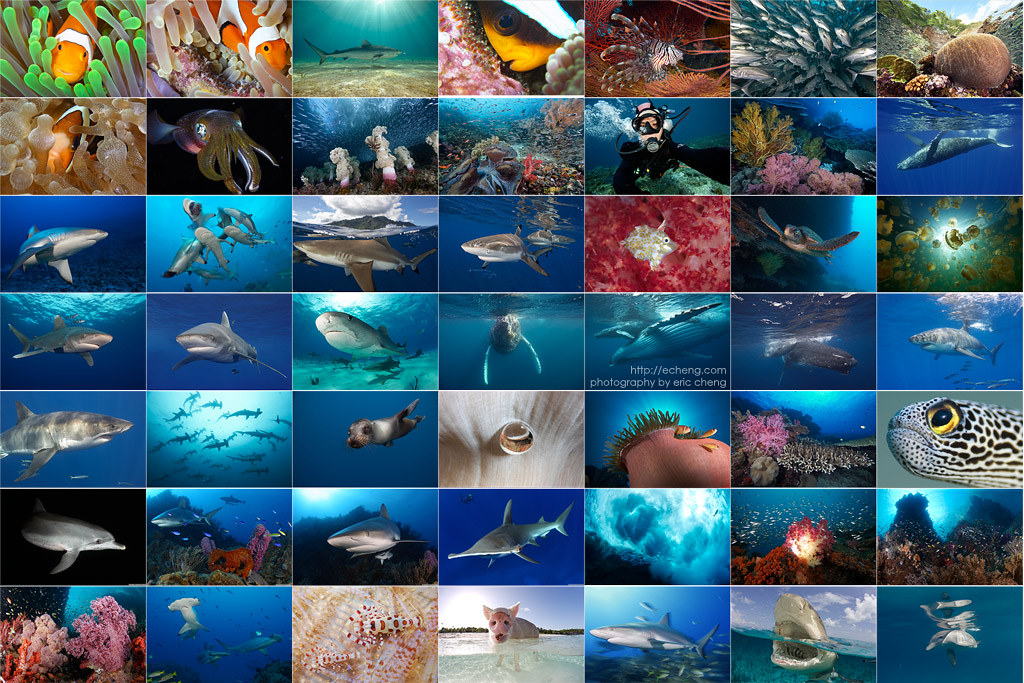This collage features an underwater theme with a total of 56 vibrant images showcasing an array of marine life and ocean scenes. Arranged across multiple rows and columns, the majority of the images capture various species of sharks, which are the most frequently depicted. The top row includes three pictures of clownfish, differentiated further by an additional one in the second row. Interspersed throughout the collage are images of a scuba diver seemingly taking a selfie, a playful pig in the water, sea turtles, and various sea anemones and corals. The vivid underwater scenes highlight a spectrum of blues and bursts of red, complemented by images of green algae and other aquatic plants. Among the diverse marine creatures, there's also a solitary dolphin, a couple of hammerhead sharks, and either an octopus or squid, enriching the dynamic representation of ocean life in this visual collection.